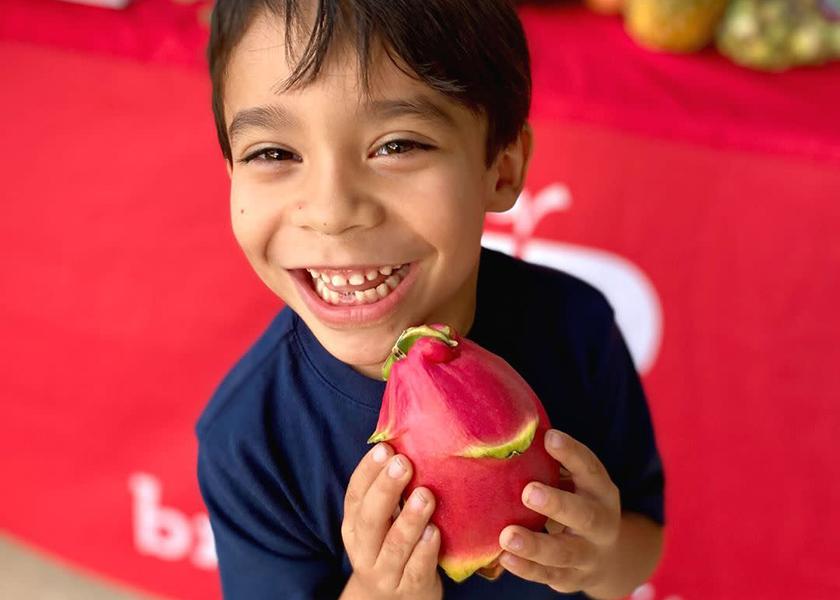In this color photograph, a happy young boy with brown eyes and dark brown hair is smiling brightly, revealing a gap where two of his bottom teeth are missing. He is wearing a blue t-shirt and holding a dragon fruit with both hands. The dragon fruit, characterized by its pinkish-red skin and yellowish-green scaly wings, stands out prominently as the main object in the image. The background features a red tablecloth and other indistinct items, possibly fruits, with vague white lettering that is difficult to discern. The boy's joyful expression and the vibrant details of the dragon fruit create a captivating and heartwarming scene.